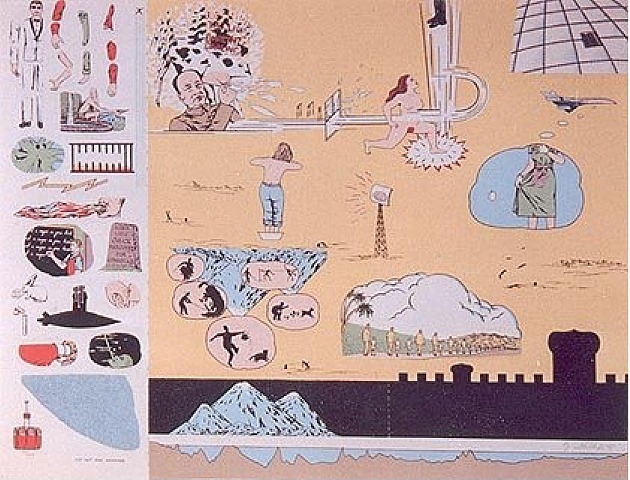The image is a detailed, hand-drawn, computer-generated artwork with a comedic flair, featuring a peach and light pink background. On the left-hand side, there's a series of random, segmented body parts and smaller pictures, including a man writing on a blackboard, a couple atop a black submarine, and a man in a white suit. Among these, there's also an unusual rabbit seemingly smoking. 

In the top scene, a man is milking a cow, adjacent to a naked woman stepping on another person's toe, causing him to jump high enough that only his boots are visible. To the right, there's an airplane with a thought bubble depicting a woman checking her stained dress. Lower in the image, over a purple foundation gradually blending into a beige backdrop, there is a mixture of structures and landscapes, including the shadow of a castle wall, mountains, and an inverted mountain with a man playing with his dog, surrounded by thought bubbles. 

The entire composition mimics an action cartoon, peppered with odd shapes, buildings, and animals, giving it an eclectic and visually engaging impression.